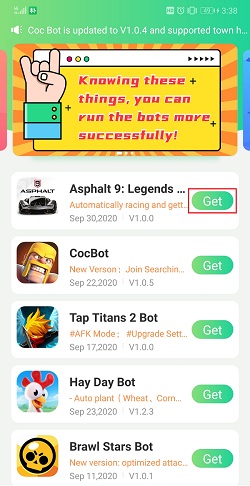A detailed caption for the described image would be:

"A screenshot of a web page displayed on a cell phone is shown. At the top of the screen, the status bar indicates the cellular signal strength on the left side, while a square icon with 'HD' in capital letters is positioned on the opposite side. Next to the HD icon, there is an alarm clock symbol, followed by the battery icon indicating it is charging at 49%, and the current time shown as 3:38.

Below the status bar, the main content features a speaker icon paired with the text 'Cookbot is updated to V1.0.4 in supported town.' Embedded within this section is a graphic with horizontal stripes in shades of orange, and a cartoon hand making a peace sign with the pinky and forefinger raised.

The top banner is white with a traffic light-like red, yellow, and green circles. The header text reads, 'Knowing these things you can run the bots more successfully.' 

Underneath the banner, there are five distinct options listed against a white background: 'Asphalt 9: Legends,' 'Cookbot,' 'Tap Titans 2 bot,' 'Hay Day bot,' and 'Brawl Stars bot.'"